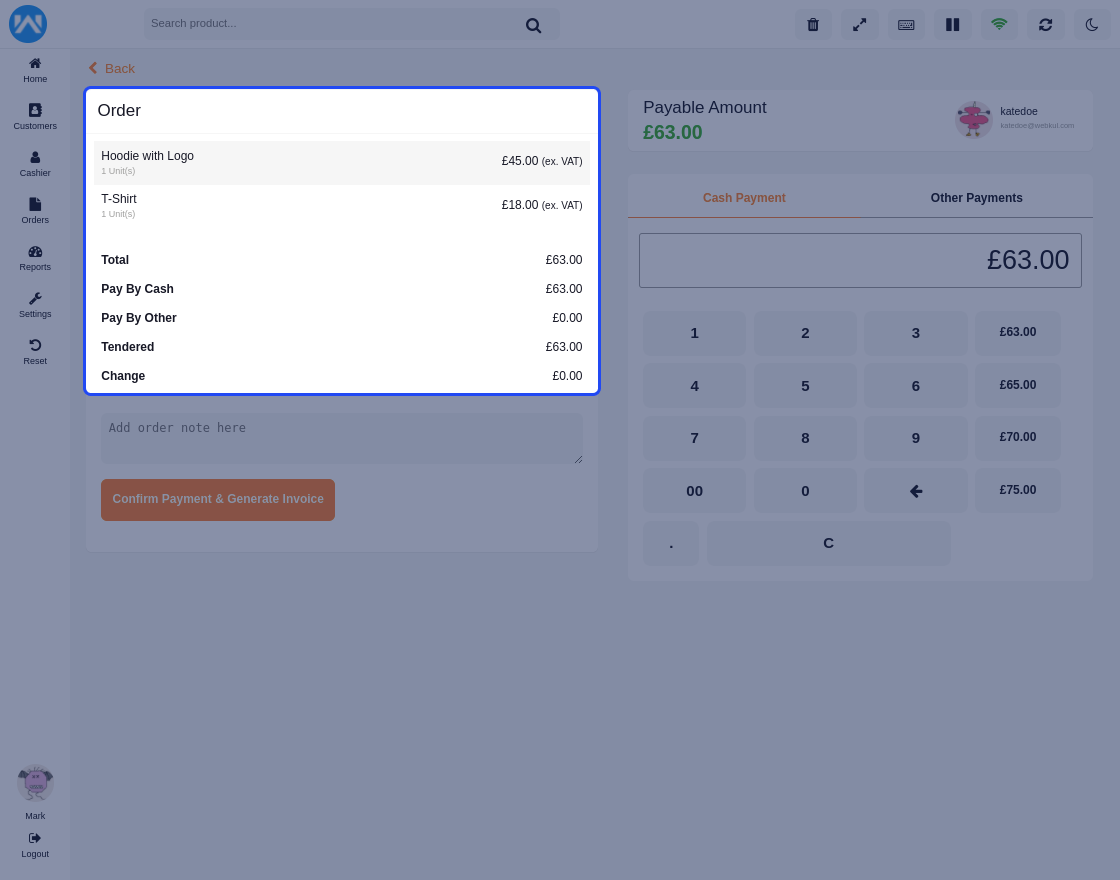The image shows a rectangular pop-up window with a light grey background on a slightly bluish-grey screen. The pop-up has a faint blue outline and contains various financial details. On the left-hand side, in black text, it says "Order" followed by "Order with Logo". Next to this text is a Euro sign (€) with the amount 45.00, followed by "EX.VAT". Below this, it lists "T-shirt", another Euro sign for 18.00, and "EX.VAT" in front of it. Underneath these items, the pop-up displays a summary in black text, stating "Total. Paid by Cash. Paid by Other Tender Change." On the right-hand side, it shows amounts in Euro: 63.00, 63.00, 0.00, and 63.00 respectively.

Towards the bottom of the pop-up window, it reads "Payable Amount" in black, with a Euro sign (€) and 63.00 in green beneath it. There are two tabs below this section: an orange underlined tab that says "Cash Payment" and a black tab labeled "Other Payment." Under these tabs is another rectangular box outlined in black, containing the Euro sign (€) and the amount 63.00.

At the very bottom of the pop-up, there is an integrated calculator with all the basic numbers, each displayed within its own small box with black text.